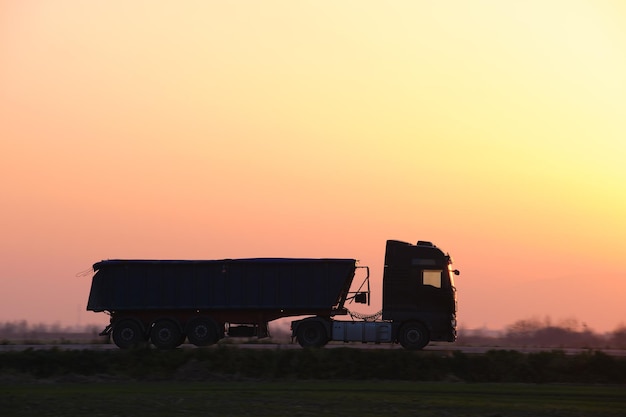In the photograph, a large dump truck with a flat front and multiple axles is prominently positioned, facing the right side of the frame. The truck's substantial tires and open pickup area are silhouetted against a captivating sunset or sunrise sky, which transitions from a brilliant yellow at the top to vibrant shades of orange and pink closer to the horizon. The road on which the truck travels appears narrow and possibly rural, partially obscured and barely visible underneath. Below the road, a green grassy field provides a lush contrast. In the background, the horizon is dotted with the faint shapes of either building-like structures or trees, enhancing the solitary and expansive feel of the scene.